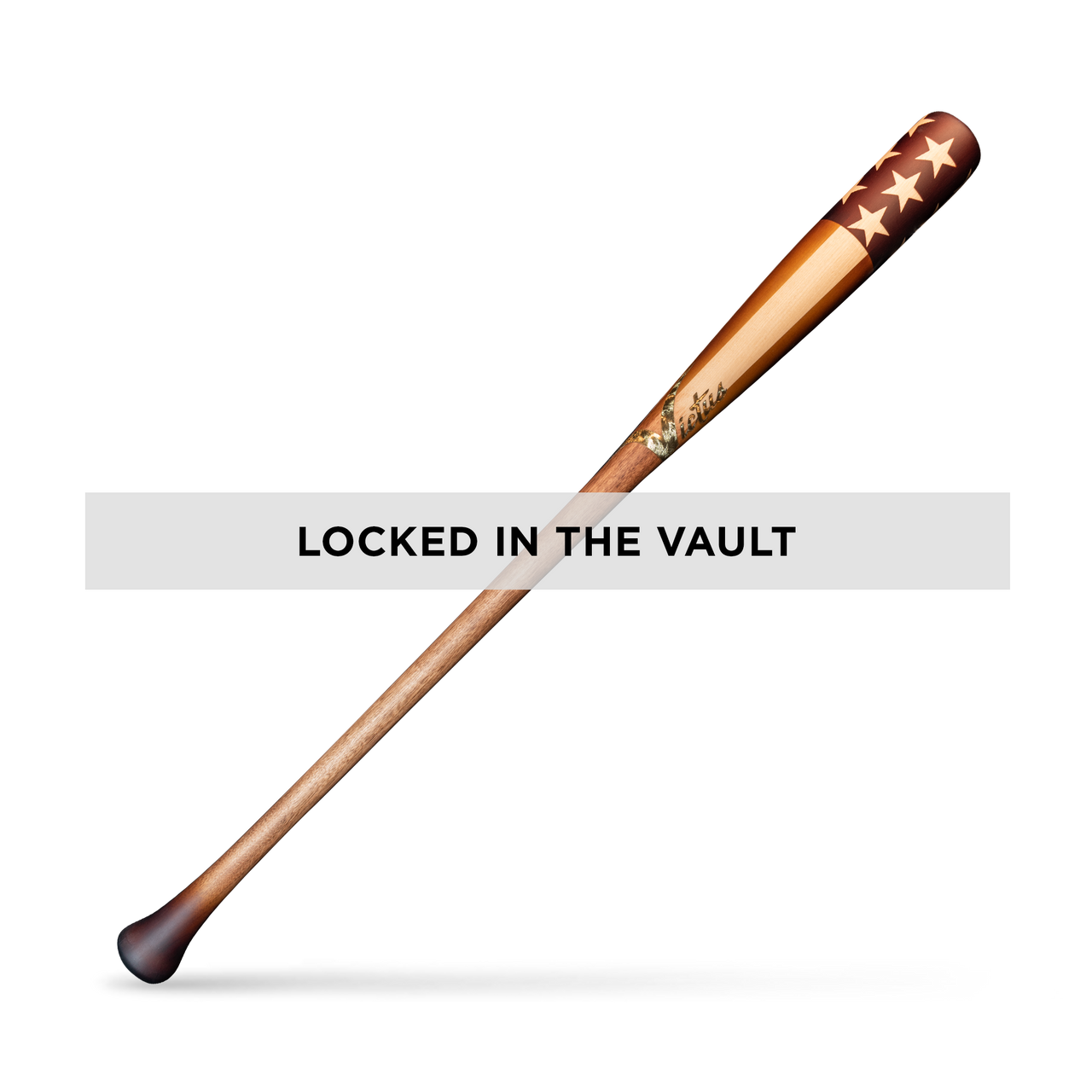The image depicts a wooden baseball bat laying diagonally against a solid white background. The bat's knob at the bottom left corner is darker brown, transitioning to a lighter brown towards the barrel. The tip of the barrel at the top right corner features a design resembling the American flag, with red and white stripes, and three white stars on a blue background. The word "Victus" is scripted within this flag-like design. Additionally, the bat has an overlaid gray rectangle across its length, within which the words "LOCKED IN THE VAULT" are written in bold black letters. This combination of patriotic imagery and text creates a striking visual contrast against the white background.